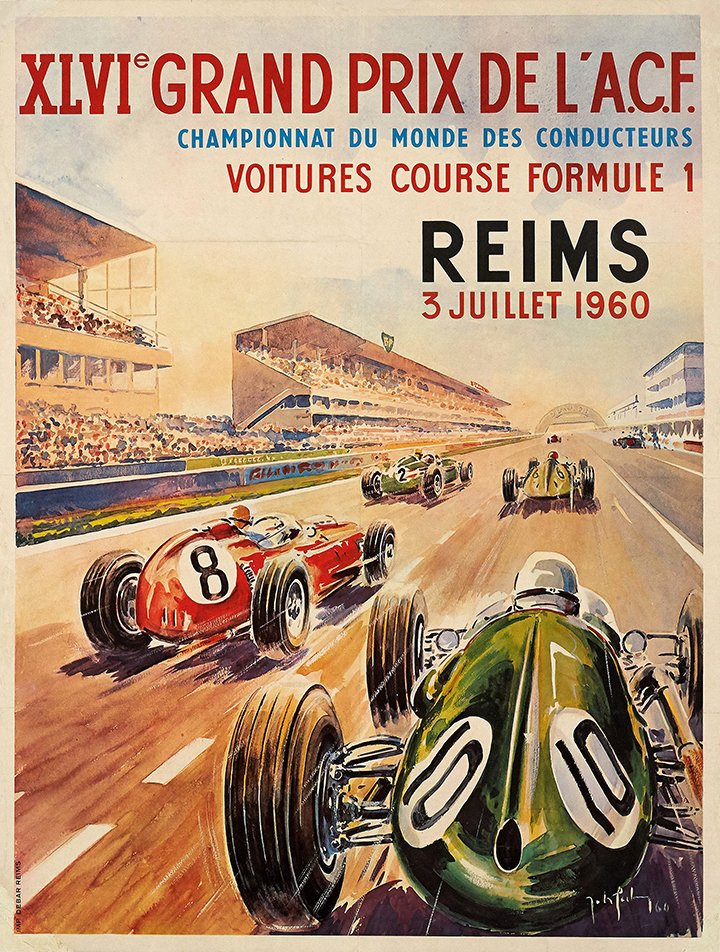The Illij is a vintage-style promotional poster for the Championnats du Monde des Conducteurs, featuring an all hand-drawn and painted depiction of a Grand Prix race that took place on July 3, 1960. The artwork showcases multiple old-style racing cars, with numbers such as 8, 10, 2, and 6, racing away from the viewer towards a distant archway. The scene captures the dynamic energy of the race, set on a two-lane road with a white dotted line in the center. On the left side, the crowd is represented by various dots in a raised seating area, while the right side features blocky buildings, likely additional observation decks or seating areas. The cars themselves are cylindrical, low to the ground, attached to silver-colored suspensions, with small view screens for the drivers. The title of the poster is rendered in a combination of red and blue letters, and the artist has signed their name in white ink at the bottom of the image.